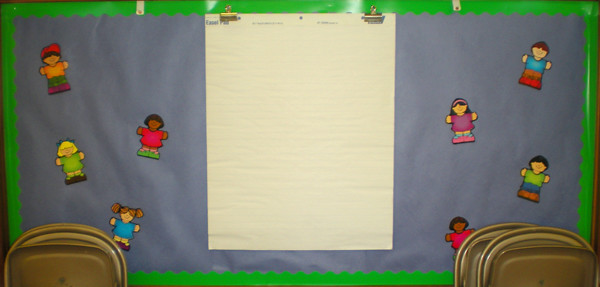The image depicts a decorated bulletin board typically found in an elementary school setting. The bulletin board features a vivid blue paper background bordered by a wavy, lime-green paper trim. Affixed to the blue background are eight colorful paper cutouts of children, each adorned in varied outfits including shades of blue, green, pink, orange, purple, and brown. Notably, one of the boys is wearing a ball cap, while another child sports a purple dress. In the middle of the board, two small bronze-colored clips hold a large white poster that appears to have exam-like content, though the details are hard to discern. Adjacent to the bulletin board, there are three or four folded metal chairs neatly stacked against the wall. The board itself is secured to the wall by two visible metal brackets at the top. The entire setup evokes a cheerful and educational ambiance commonly seen in school environments.